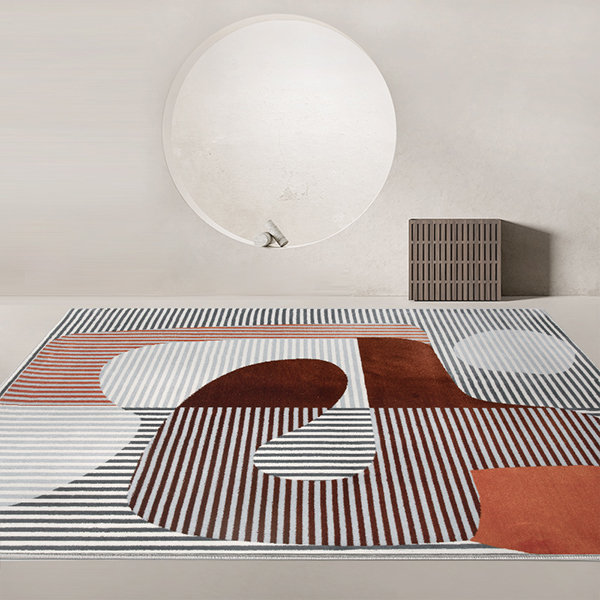In the image, we see a minimalist white room with both the floor and wall painted in a stark white hue. The centerpiece features a circular disc that might be a decorative alcove or a mirror. Positioned centrally within this alcove are two small objects resembling rolled-up towels, adding a subtle element of texture.

Dominating the lower part of the image is a large, abstract placemat or rug, characterized by an intricate patchwork of black-and-white striped lines arranged both horizontally and vertically. The design is further complicated by additional lines, circles, and half-circles that create an eclectic mix of patterns with no clear symmetry. To the right of the central disc, there's a square-shaped piece of furniture, possibly wooden, with grayish-brown slats running horizontally. The overall aesthetic of the room is stark yet dynamically detailed, creating an intriguing visual contrast.